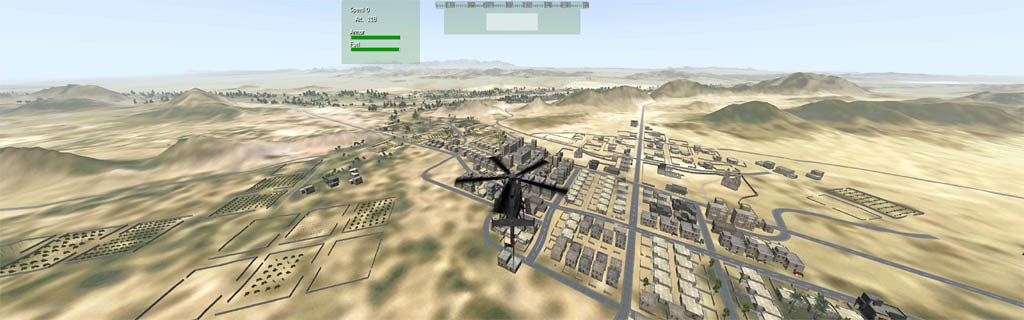This screenshot from a video game, characterized by its low graphical fidelity, presents an expansive, rectangular landscape. The image, notably wider than it is tall, captures an aerial view of a desert cityscape. The sky dominates the top portion and is a pale, cloudless blue. In the center, a black helicopter with an indistinct cargo dangles below it hovers over the city laid out in a grid. Rows of identical brown, gray, yellow, and green-colored buildings and factories, interspersed with thick gray roads, stretch across the landscape. At the top, two green boxes contain blurred, illegible information, each featuring green bars, possibly indicating stats like health or progress.